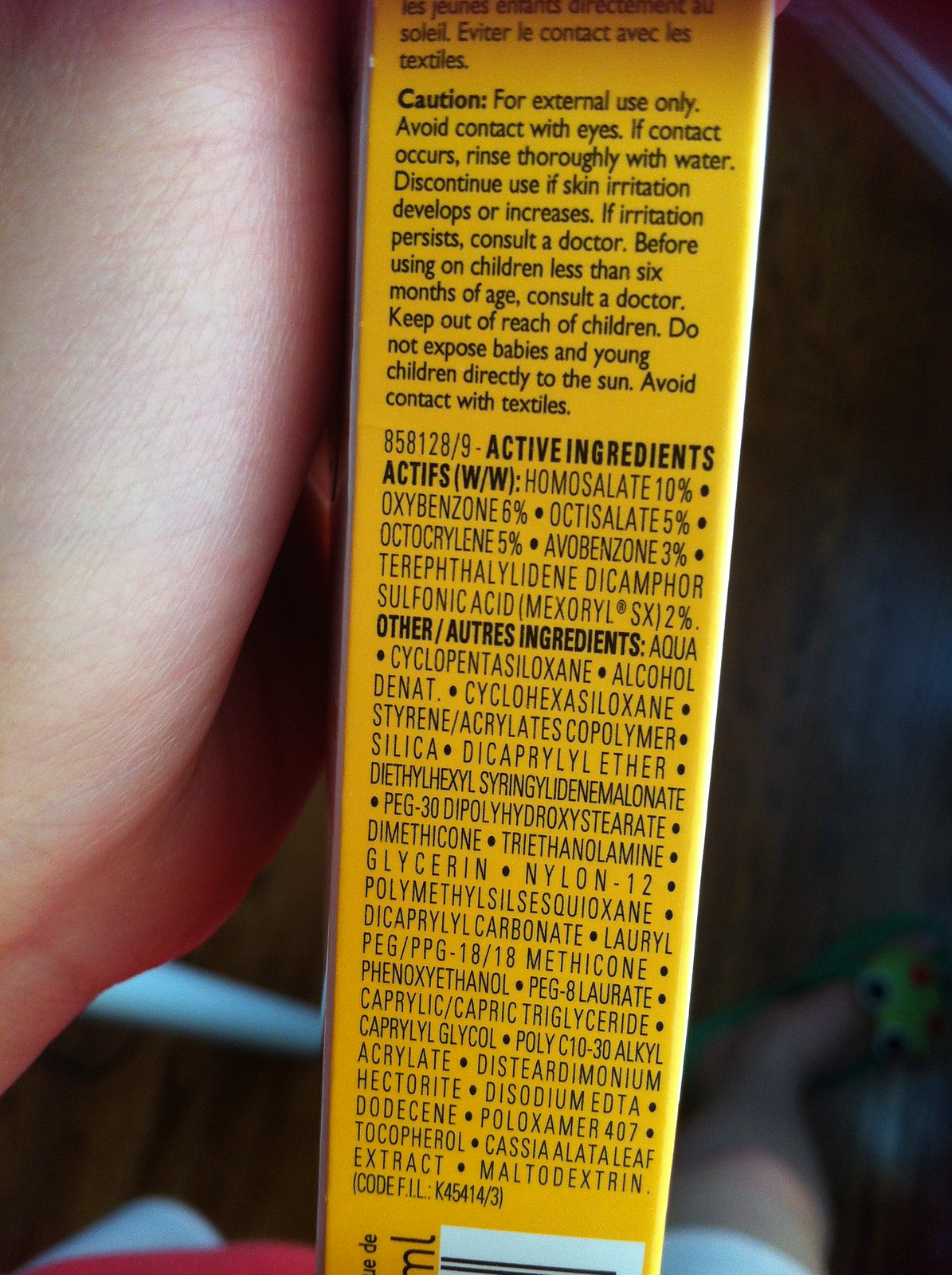This close-up photograph captures the side of a yellow box being held by a person. The person's hand, prominently featured, displays fine details such as pores and the intricate lines of the skin. The image focuses on the thumb and part of the palm, with no fingers visible. The individual, wearing red attire, is lightly tanned and standing on a wooden floor. They are also spotted wearing a green flip-flop. Part of a leg is visible in the foreground. The box features cautionary text, warning against external use and advising to avoid contact with eyes, keep out of reach of children, shield young children from direct sun exposure, and avoid contact with textiles. A segment of a barcode and the letters "ML" are partially visible at the bottom of the box. In the background, the white molding of the room adds a subtle context to the setting, which is presumed to be within a home.